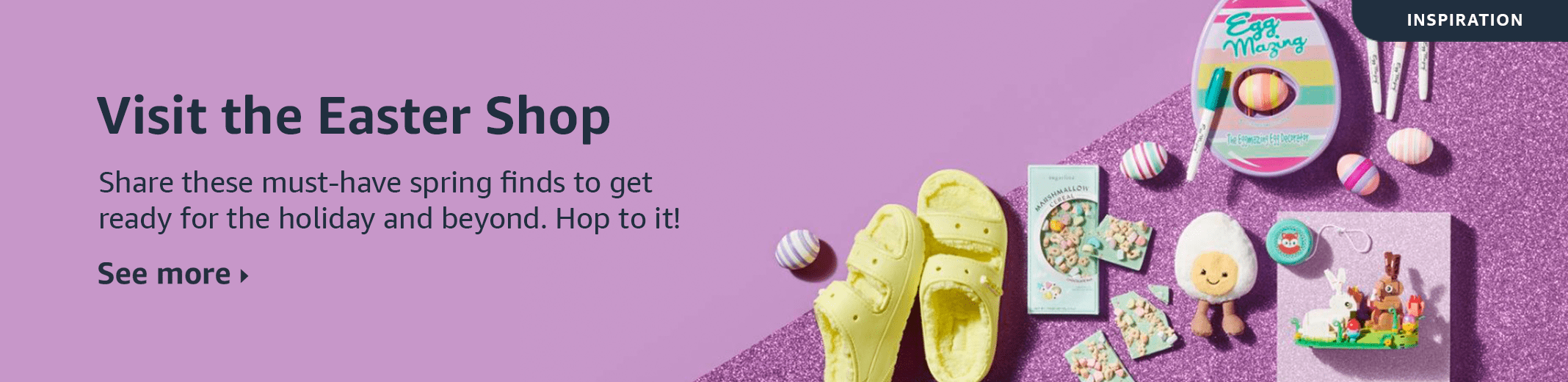**Easter Shop Banner on Shopping Website**

The banner showcases a vibrant, pastel-themed Easter Shop section of a shopping website, set against a lilac-purple background. To the left, black text greets viewers with the message, "This is the Easter Shop. Sure, these must-have spring finds to get ready for the holiday and beyond. Hop to it!" followed by a tiny arrow encouraging users to explore further.

In the upper right-hand corner, a black, curved rectangle bears the word "Inspiration" in white. A diagonally textured section, resembling a sandy surface, slices through the right side of the background, seamlessly integrating with the rest of the design.

Various Easter-themed objects adorn the textured area, some spilling over slightly onto the smoother portion of the background. These include at least four striped Easter eggs, a pair of yellow sandals, and a card decorated with eggs. There's also a charming little cartoon figure with a yellow face and legs, resembling a half-boiled egg. Among the scattered items are a larger striped egg nestled within a smaller egg, and a couple of Easter cards each featuring bunnies with prominent shadows beneath them.

Additionally, the upper left part of the diagonal section displays a pale violet circle, while a pale bluish card occupies the left side. Just beneath the "Inspiration" logo, to the upper right, a set of pens is neatly positioned, completing the festive and detailed presentation.